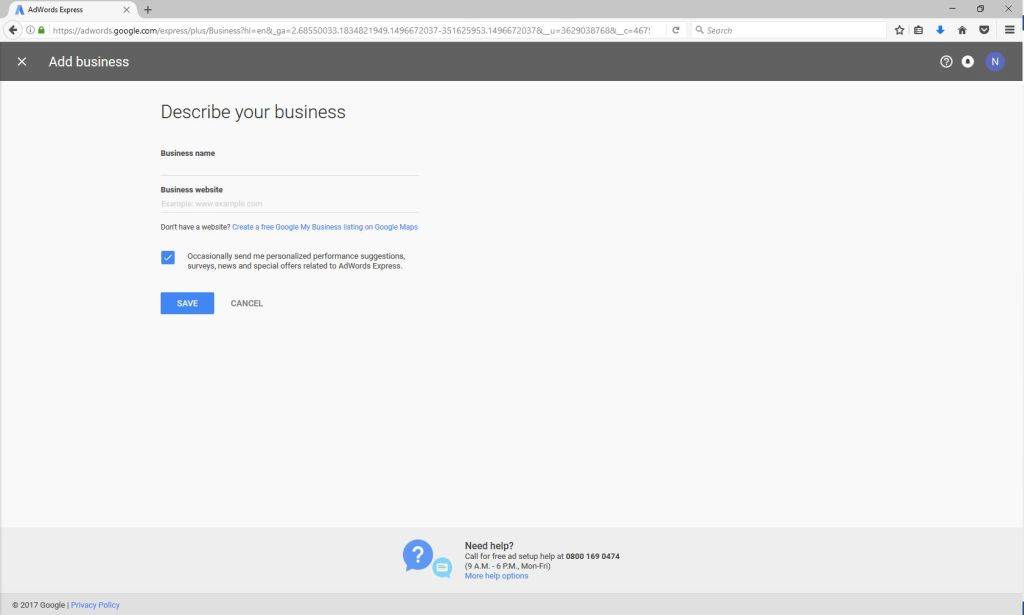The image showcases a webpage from Google AdWords Express. The browser page header displays "AdBusiness" in white text on a grey background in the top left corner. To the right of the header are a white question mark icon and a blue circle with a white "N". 

The main content area consists of a form with a white background and black text, prompting the user to "Describe your business". The form includes fields for "Business name" and "Business website". Below these fields, there is an option to "Create a free Google My Business listing on Google Maps", written in blue text.

Underneath, a checked blue checkbox labeled "Occasionally send me personalized performance suggestions, surveys, news, and special offers related to AdWords Express" is visible. Below the checkbox are two action buttons: a blue "Save" button and a grey "Cancel" button.

At the bottom of the page, it reads "Need help? Call for free ad setup help: 808-001-690-474". Next to this, there is a blue textbox with a white question mark symbol, and another icon featuring a light blue circle with a white letter "N". Additionally, there's a "More help" option written in blue text.